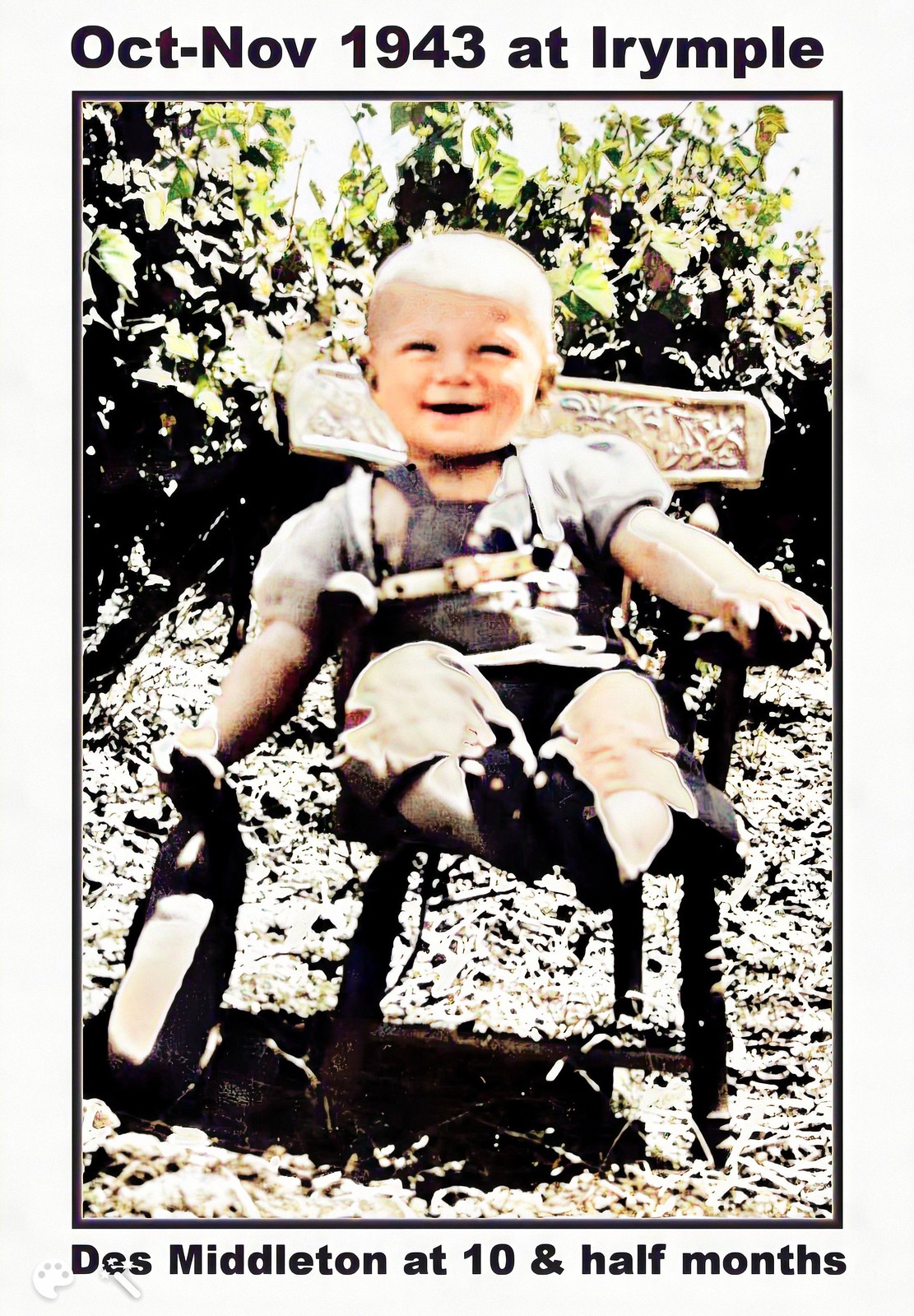This black-and-white photo from October-November 1943, taken at Eryimple, features a young child identified as Des Middleton at 10 1/2 months old. Des is seated in a small black chair with a tan upper back, appearing to be strapped in with a belt-like strap across his upper body and shoulders. He sports blonde hair, a big smile, and is wearing blue overalls over a gray t-shirt. His right hand extends below the chair, holding an object—possibly a stuffed animal or a bag of something black and white—that touches the ground. Des’s left hand rests on the arm of the chair. The scene is set outdoors with green shrubbery and dry grass or dead leaves visible behind him and around the chair. The caption above the photo reads, "October-November 1943 at Eyrimple," and below it states, "Des Middleton at 10 1⁄2 months."